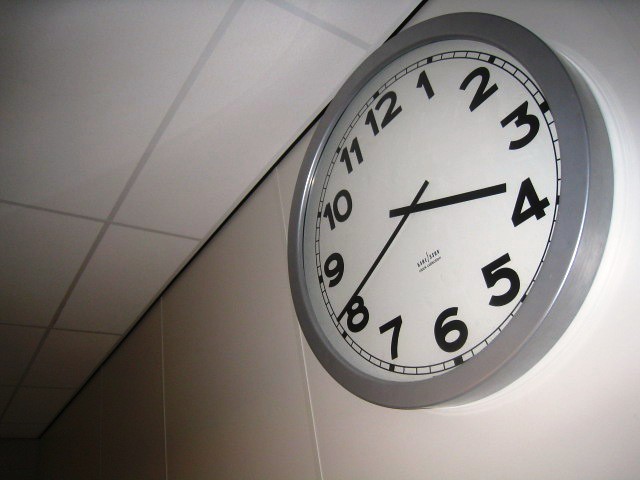A close-up view of a round wall clock mounted high on a white wall, close to the ceiling. The clock features a sleek silver outline, accentuating the minimalist design of the white dial face. The numerals, along with the hour and minute hands, are in bold black, ensuring clear legibility. Positioned above the number six is the clock's brand, presented in two lines of text, though they are not legible even upon closer inspection. The time displayed on the clock is 4:41. The room's walls and ceiling are painted a pristine white, with subtle gray lines running both horizontally and vertically, adding a touch of texture to the otherwise clean and simple decor.